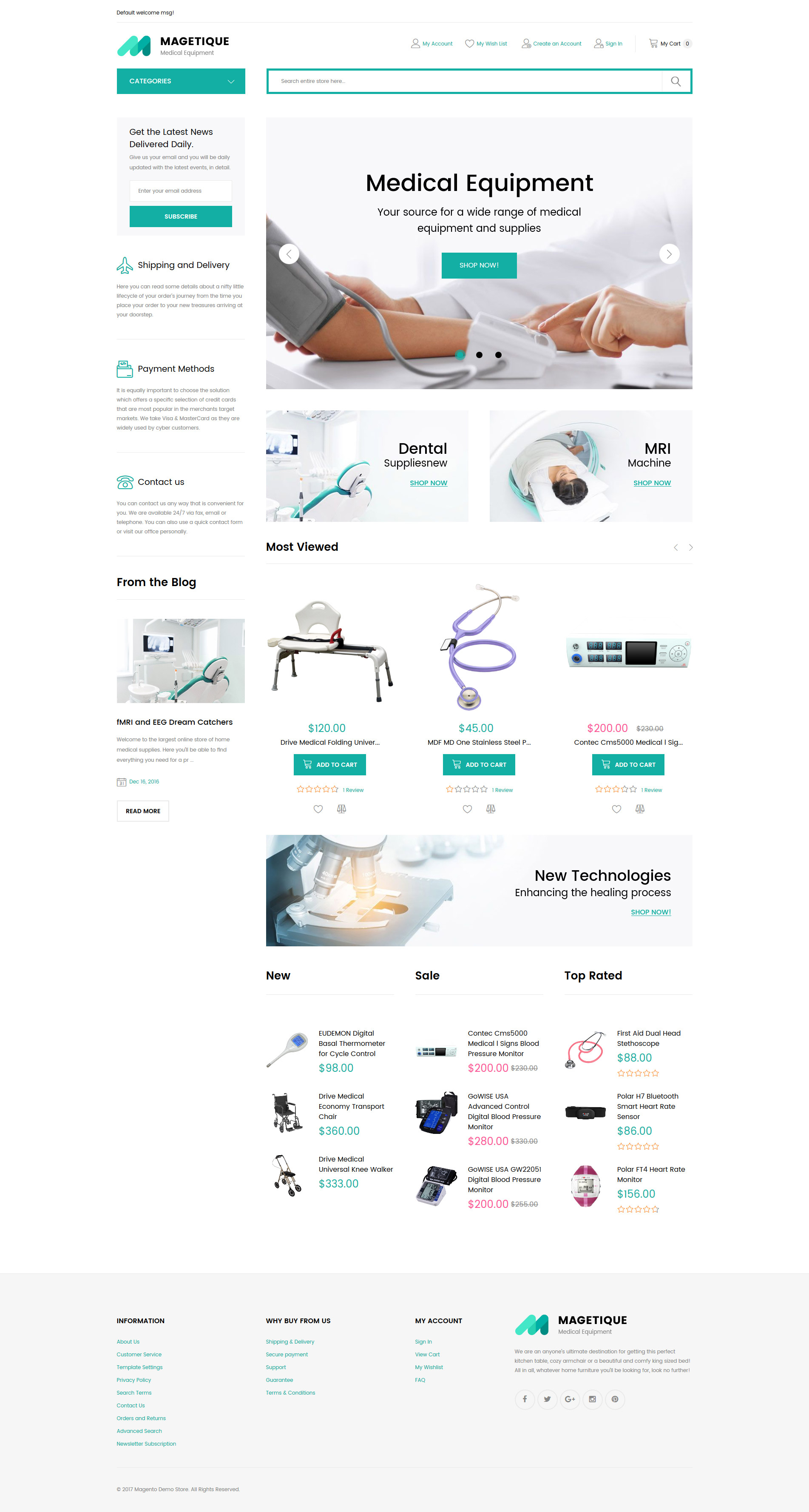The image captures a vertically elongated web page dedicated to medical equipment. The web page belongs to a company or site, the name of which is located at the top left corner. Adjacent to the company's name, towards the right, is a search field highlighted with a teal green outline. Directly below this, a prominent image depicts an arm extending from the left side of the frame, fitted with a blood pressure cuff. An arm clad in a lab coat extends from the right side, engaging with the equipment.

Central to the image is the heading "Medical Equipment: Your source for a wide range of medical equipment and supplies." This is immediately followed by two smaller, side-by-side images labeled "Dental" and "MRI." As the viewer's eye moves downward, they encounter a series of item listings that progressively decrease in size. These listings are accompanied by corresponding images and brief descriptions.

At the very bottom of the page, there are three rows, each containing three small listings, providing further details on various products. On the left side, beneath the company's name, a vertical list appears, likely containing articles or additional information. Among the readable entries are "Payment Methods" and "Contact Us."